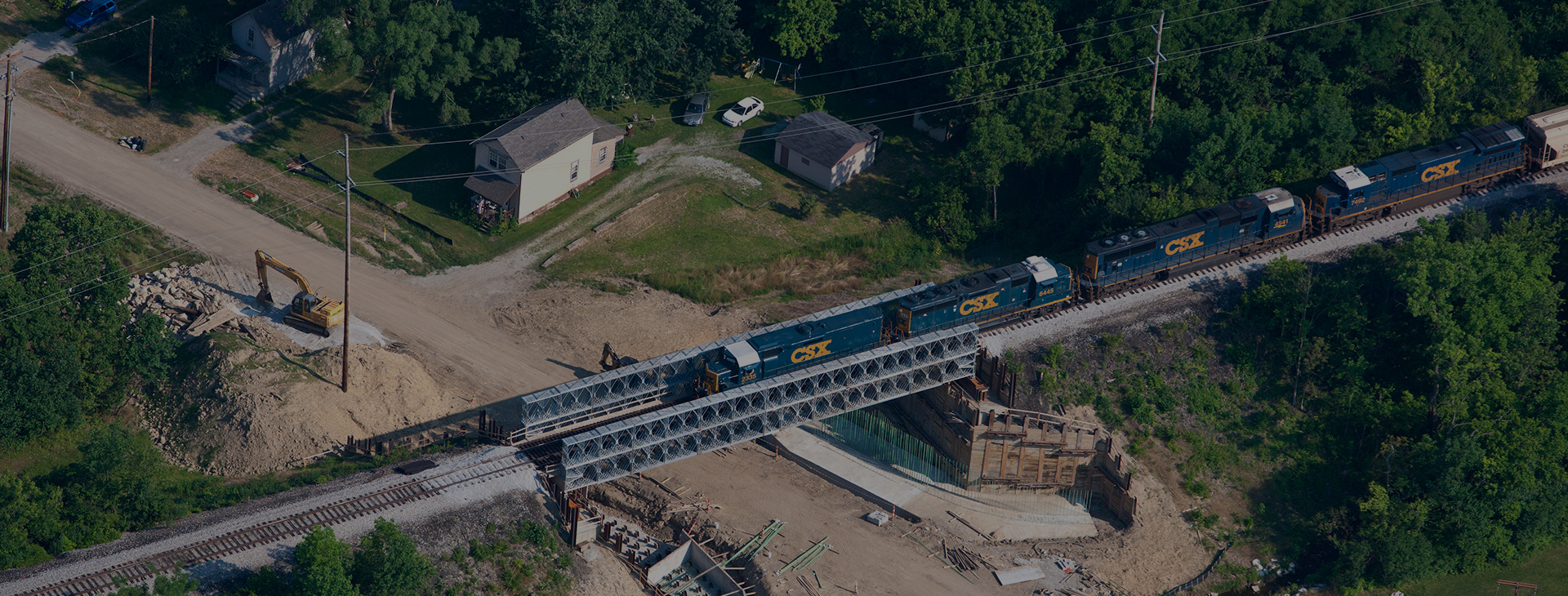This aerial photograph offers a sweeping view of a sprawling construction site interwoven with a verdant forest. The central focus is a straight, silver metal bridge supporting a dark blue CSX freight train with four carriages prominently marked in yellow. The train traverses the image diagonally from bottom left to top right, emerging from a lush wooded area and crossing over an actively worked dirt road. Below the bridge, the road, in the midst of construction, leads into a sparse residential zone characterized by three houses with gray roofs and a scattering of sedans parked on the grass. Adjacent to this, there's a dirt mound atop which sits a yellow construction vehicle, engrossed in the site's development. The structural simplicity of the bridge contrasts with the dynamic natural and human activity surrounding it, encapsulating a moment where industry and nature converge.